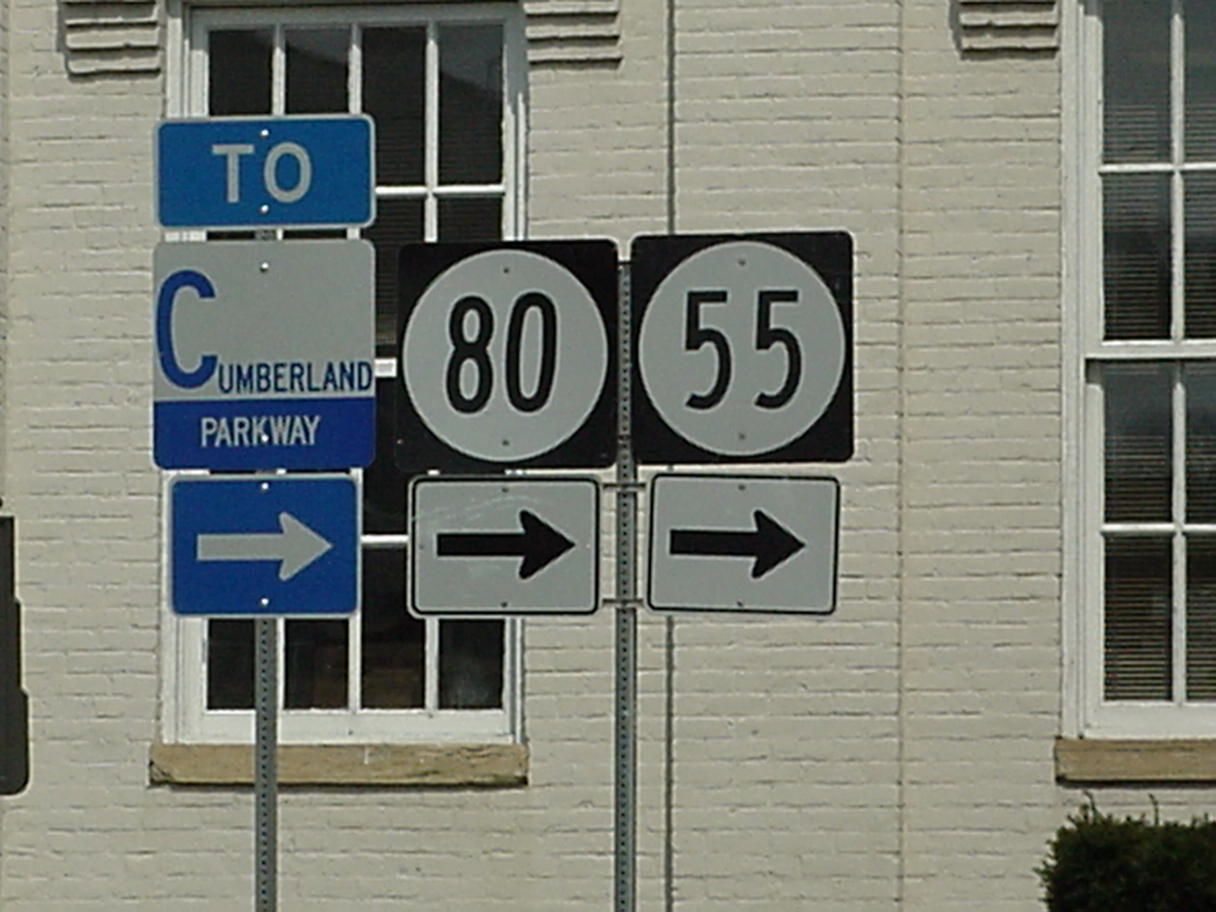This image captures a cluster of directional highway signs situated at what appears to be a stop sign, guiding traffic towards the right. The scene is set in front of a historic-looking brick building adorned with multi-pane windows and a well-trimmed hedge. The signage includes an oval black sign with white numbers for Highway 80 and Highway 55, each featuring a right-pointing arrow. Additionally, there's a blue and white sign indicating the route to Cumberland Parkway, also directing to the right. A series of poles hold these signs: one pole displays three signs while another has four, all collectively emphasizing the rightward direction. The setting is outdoors, with the signs standing out clearly against the backdrop of the aged architectural structure.